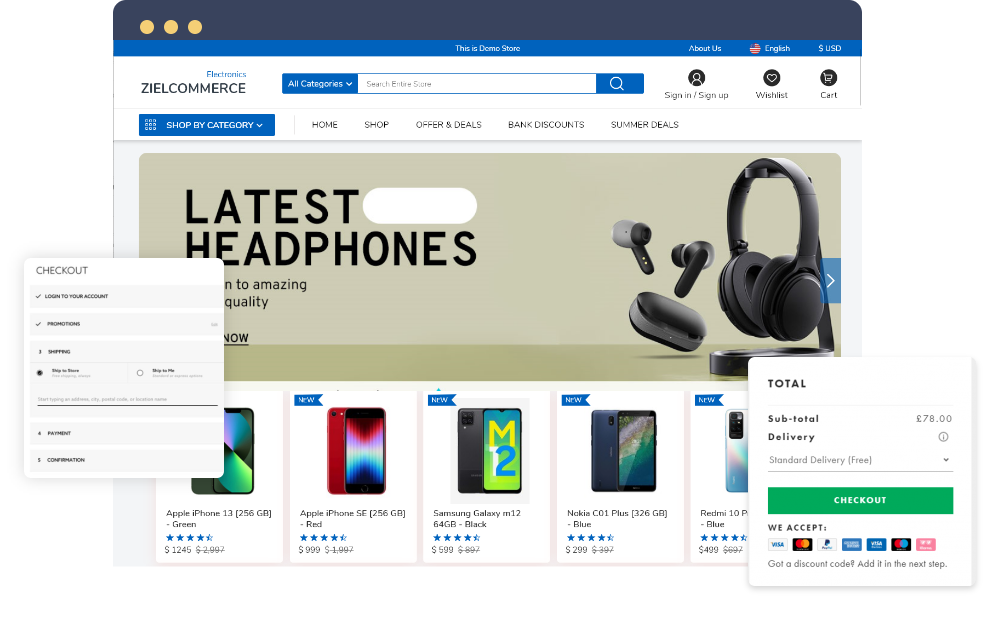The image depicts the homepage of a demo e-commerce website named "Ziel Commerce." At the top of the page are three beige dots set against a blue background. Below this section lies a royal blue navigation bar featuring centered text that reads "This is a demo store." To its right are links for "About Us," a language selection dropdown with an English (United States) option, and a currency selection set to U.S. dollars.

Directly to the right of the website's name, "Ziel Commerce," is an "All Categories" dropdown, followed by a search bar. Further to the right are links for "Sign Up/Sign In," "Wishlist," and "Cart."

Beneath the navigation bar is a menu listing categories such as "Home," "Shop," "Offers and Deals," "Banks and Discounts," and "Summer Deals." The main image in the center showcases a pair of black wireless earbuds with stems, a charging case, and headphones, along with a checkout dialog box on the left side. This overlay includes options to log into your account, view promotions, and proceed through shopping, payment, and confirmation steps.

In the lower section, the page displays various Apple iPhone models currently available for sale, including the iPhone 13. Each phone listing provides a rating, storage capacity details, the MSRP, the current selling price, and offers for three other phones. At the bottom, a summary box shows the subtotal, delivery cost, accepted payment methods, and a prominent green "Checkout" button.